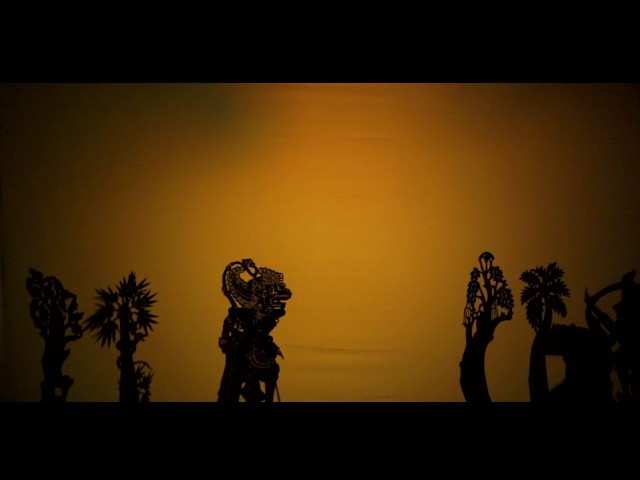The image depicts a dramatic scene reminiscent of a shadow puppet show, featuring shadowy silhouettes set against a cloth background illuminated in a golden-orange hue. The light is concentrated in the center, creating a glowing effect, while the corners descend into darkness, emphasizing the central figures and adding depth to the overall composition.

In the middle of the scene, slightly to the left, stands a prominent figure with the distinct appearance of a Chinese lion statue combined with the burly body of a soldier, held upright potentially by a rod at the bottom. This central character is flanked by a variety of silhouetted trees. On the left side, the trees include one with rounded, chili-shaped leaves and another with spiky foliage, suggesting diverse tropical influences. On the right, there are trees with grape-like clusters of leaves and short spikes.

Beneath these botanical forms and to the lower right, there's an indistinct object, shrouded in shadow, making it difficult to identify. Despite the enigmatic narrative, the scene suggests a lively storytelling tradition, possibly rooted in Malaysian culture, given the stylistic elements and figures depicted. The silhouettes appear strikingly two-dimensional, with a slightly uncanny, almost computer-generated quality, enhancing the mysterious and enchanting atmosphere of this visual tableau.